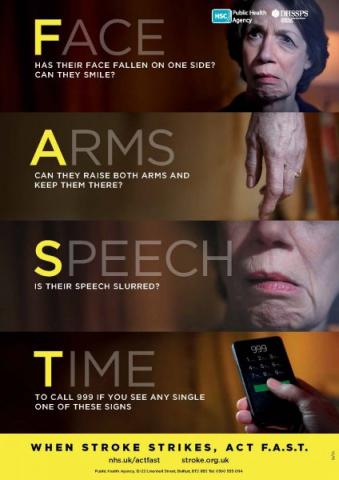The poster serves as a public safety announcement about recognizing the signs of a stroke, labeled "FAST" vertically in prominent yellow letters against a dark, multi-toned brown background. It features four key sections, each with a photograph to illustrate the associated symptom. At the top is "FACE," with an image of an older woman whose face appears to have drooped on one side. Below this, labeled "ARMS," is a photograph of her trying to raise both arms. Further down, under "SPEECH," is a close-up of her mouth with discerning details that indicate slurred speech. The last section "TIME" shows a hand holding a black rectangular object resembling a phone, emphasizing the urgency of calling 999 if any of these signs are observed. At the bottom, a yellow banner urges, "When stroke strikes, act F-A-S-T," followed by an unreadable small print and a reference to stroke.org.uk.